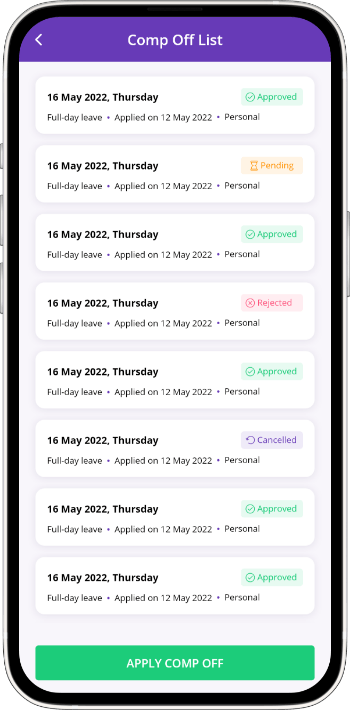The image appears to be an artist's rendering of a smartphone. The smartphone features a sleek silver border and an interface with detailed elements. On the right-hand side, there is a prominent button situated near the top of the device. Meanwhile, the left side houses three buttons; the top one being smaller than the other two.

The screen displays a user interface with a purple background. At the top, the text "Comp Off List" is prominently displayed in white. To the left of this text is a leftward-pointing arrow. 

Below this header, there are eight listed items detailed as follows:
1. **16 May 2022, Thursday** - Full day leave applied on 12 May 2022 for personal reasons. An "Approved" tag is situated in the upper right-hand corner.
2. **16 May 2022, Thursday** - Full day leave applied on 12 May 2022 for personal reasons. This entry has a "Pending" tag in the upper right-hand corner.
3. **16 May 2022, Thursday** - Full day leave applied on 12 May 2022 for personal reasons. This entry similarly features an "Approved" tag in the upper right-hand corner.
(The remaining six entries are not detailed but likely follow a similar format.)
 
Finally, at the bottom of the screen is a prominent green bar bearing the text "Apply Comp Off" in white, suggesting a call-to-action for the user.

The overall design seems to meticulously capture the essentials of a leave management interface on a smartphone, highlighting both the pending and approved leave statuses for the specified dates.